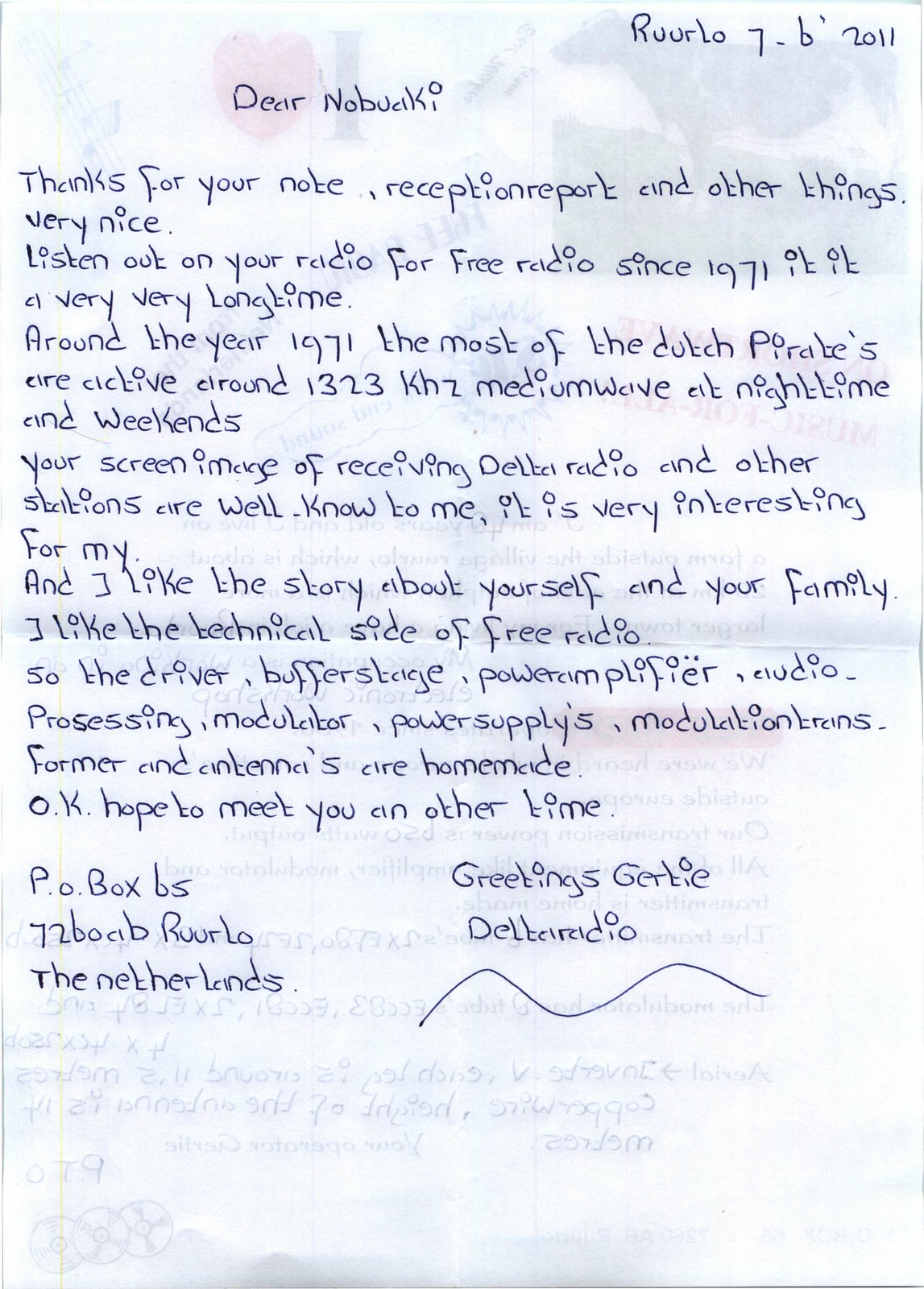The image displays a handwritten letter on white paper, possibly written on the back of another printed material as faint images of a cow and an "I ♥ something" are visible. The letter is addressed in blue ink, with handwriting slanting to the left and large circular dots above the i's, making some words hard to decipher. The upper right-hand corner of the letter contains the text "Rorlo 7-B 2011". The letter begins with "Dear Nobuaki," and continues to thank the recipient for their note, reception report, and "other things". 

The letter encourages Nobuaki to listen for free radio transmissions, which have been broadcast since 1971, mentioning that Dutch pirates were particularly active around 1323 kHz medium wave frequency during nighttime and weekends. The writer acknowledges the screen image of receiving Delta Radio and other stations, expressing interest in the technical aspects of free radio, including homemade gear like driver, buffer stage, power amplifier, audio processing modulator, power supplies, modulation transformers, and antennas.

The letter is signed, "Greetings, Gertie, Delta Radio," and provides a PO Box address in the Netherlands. The combination of personal touches and technical details creates a highly contextual and engaging letter, bridging both personal and technical narratives.